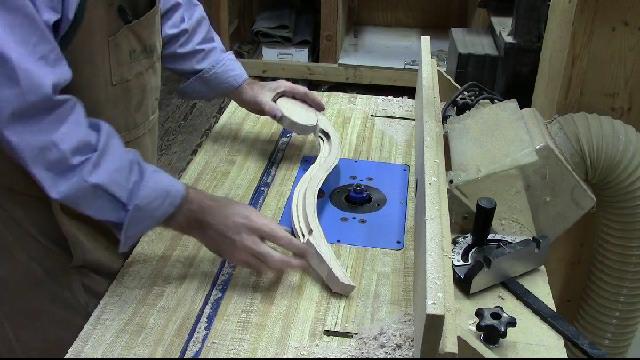In this detailed image captured from a woodworking session, a man is carefully crafting a piece of wood. Clad in a tan apron and a blue shirt with rolled-up sleeves, he demonstrates precision and skill. In his left hand, he holds a uniquely curved, circular piece of wood, while his right hand steadies it as he works. The workspace is alive with activity; sawdust is strewn across the board in the background, evidence of recent cutting. Prominently displayed in the center is a blue rectangular tool, fitted with a circular black cutting device, likely used to carve grooves into the wood, creating the visible sawdust. Behind the man, wooden shelves are neatly organized with various items, and what appears to be a PVC hose is positioned, probably intended to vacuum up sawdust. Additional tools and black knobs can be seen scattered throughout the background, completing the scene of an industrious and organized workshop.